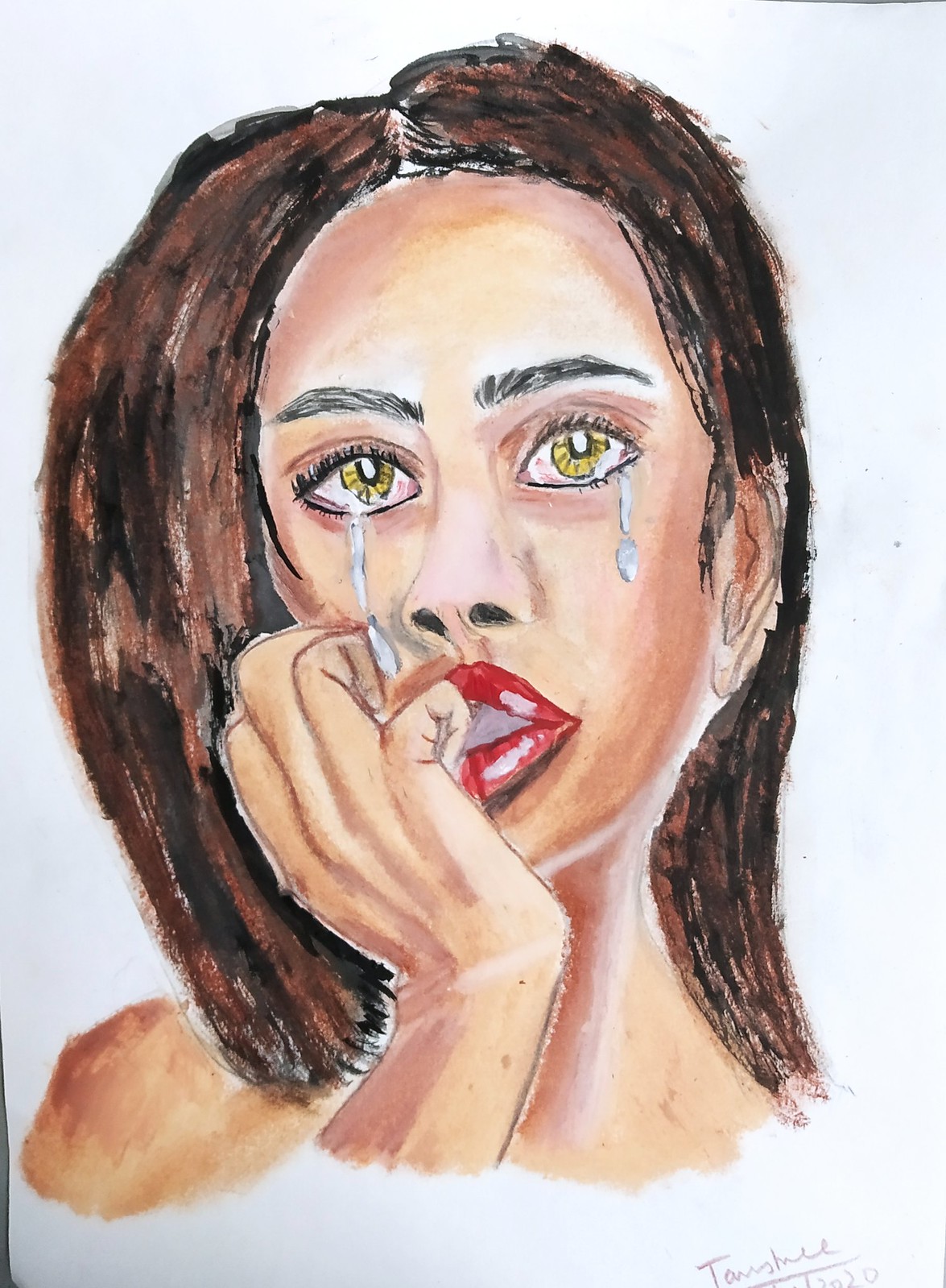This watercolor painting is a detailed self-portrait of a young woman with shoulder-length, dark brown hair. Set against a white background, the woman features well-defined black eyebrows, expressive hazel eyes accented with tears, and striking red lipstick. She appears to be in a state of worry or sadness, as suggested by her hand resting on her chin with fingers, particularly the pinky, touching her mouth, possibly indicating she is biting her nails. Her fair skin emphasizes the distinct elements of her facial expression. There is a black signature by the artist, dated January 2020, located at the bottom right corner, indicating the completion date of this remarkably well-executed artwork. The woman's gaze is directed outward, and the image captures a poignant moment, reflecting her emotional depth.